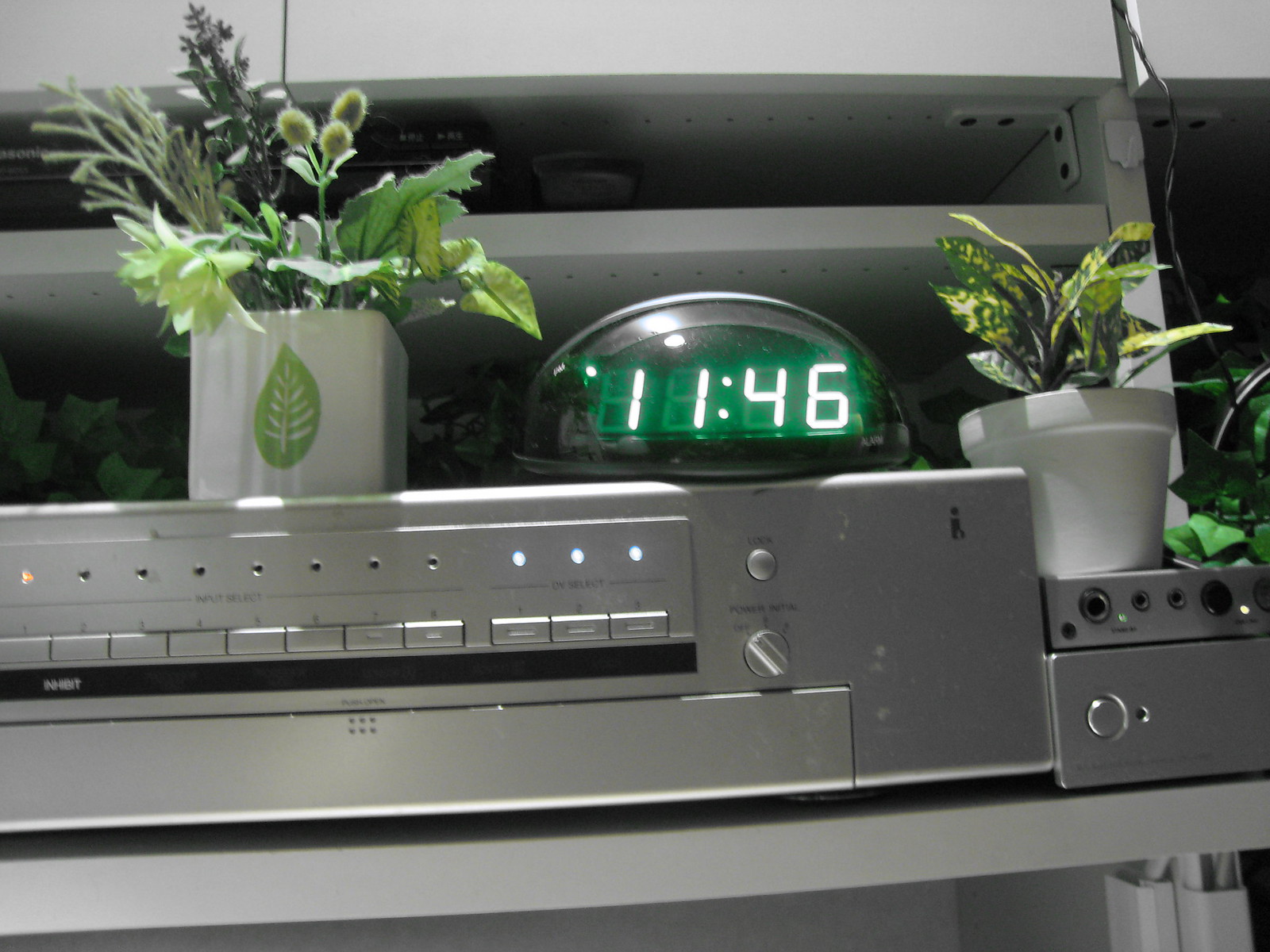The image depicts a sophisticated electronic setup comprising several components. Central to the image is a small digital clock displaying "11:46" in green digits. This clock is perched atop a long, silver electronic box that features a series of buttons and dials. The silver box is accented with black trim and a row of small indicator lights above the buttons. The majority of these indicator lights are unlit, except for one that glows yellow at one end and three that are illuminated white at the other. There are a total of eleven buttons and corresponding indicator lights, suggesting that each button has its own indicator.

Flanking the clock are two potted plants in white pots, filled with vibrant green leaves, adding a touch of nature to the otherwise technical scene. Situated beneath the long silver box is another silver device, notable for its input jacks and a solitary button next to a small, currently non-illuminated light. This entire setup is housed within a cubby of a steel cabinet, providing an organized and enclosed environment for the electronic equipment. Overall, the image captures the juxtaposition of technological precision and natural elements within a structured space.